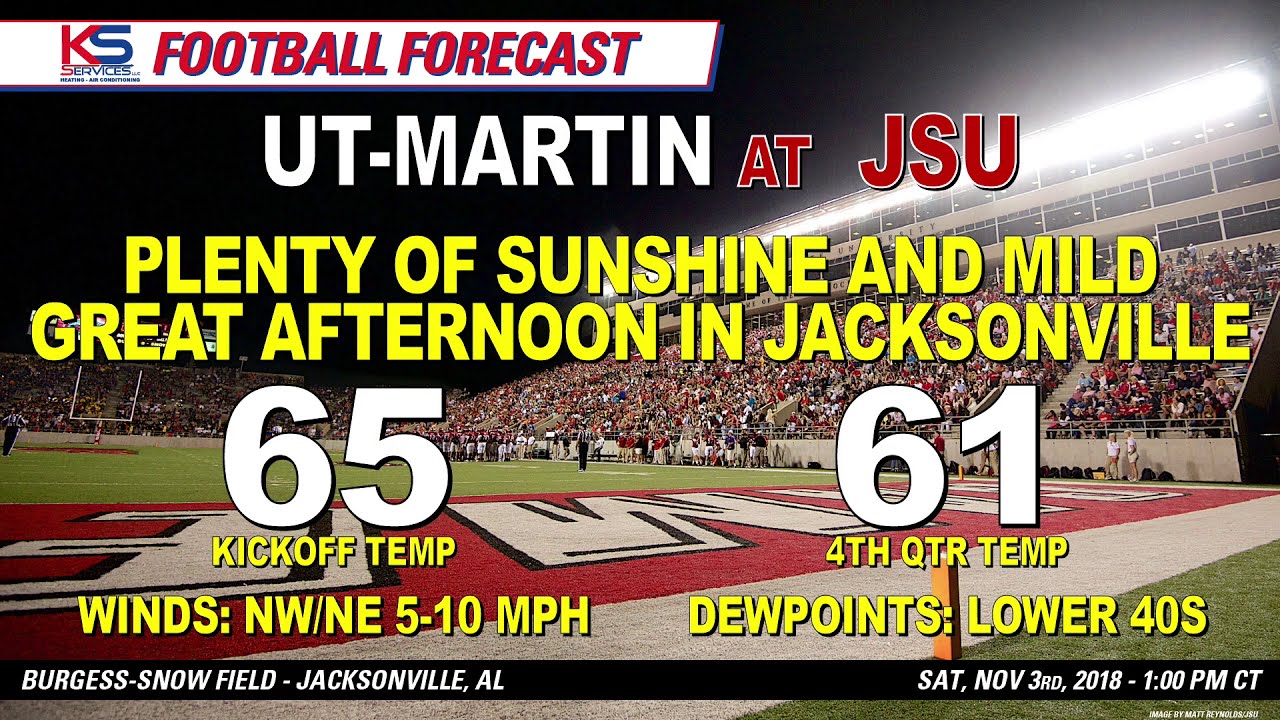The image is a screenshot of a television or monitor displaying information for an upcoming college football game, set against the backdrop of a stadium with a green field and a nighttime sky illuminated by lights. In the upper left corner, the KS Services logo is prominently displayed, with 'K' in red and 'S' in blue, followed by the words 'football forecast' in red block lettering on a white banner. Below this, the matchup 'UT-Martin at JSU' is detailed, with 'UT-Martin' in white font and 'at JSU' in red font with a white border. Additional information includes weather details in yellow font, noting 'plenty of sunshine and mild, great afternoon in Jacksonville,' with a kickoff temperature of 65°F and fourth-quarter temperature of 61°F. Winds are listed as northwest/northeast at 5-10 mph, and dew points in the lower 40s. The bottom of the screen features a black horizontal bar with 'Burgess-Snow Field, Jacksonville, Alabama' on the left side, and 'Saturday, November 3rd, 2018, 1 p.m. CT' on the right side, all in white font. The scene captures the field, a red end zone with white lettering, and a crowd in the stands under a dark sky.